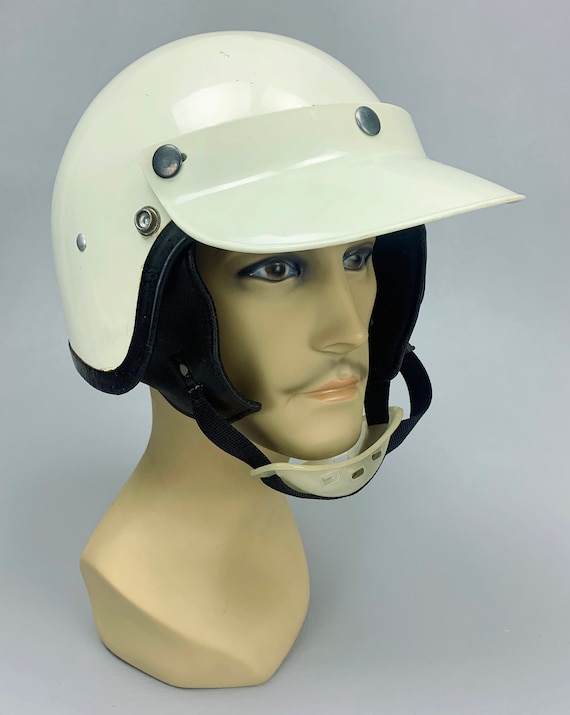The image features a close-up of a mannequin head modeled as a male with a tan complexion. The mannequin has distinctive facial features, including a long, pointy nose, brown eyes accentuated with dark black and blue eyeliner, and a faint mustache represented by a thin black line. The mannequin is adorned with a shiny, light yellow helmet with a rounded shape and a matching visor attached at the front by two silver screws. The helmet includes black flaps over both ears and a tan-colored chin guard secured by a black strap for extra protection. The background of the photograph is a solid gray, enhancing the focus on the mannequin and its detailed accessories.